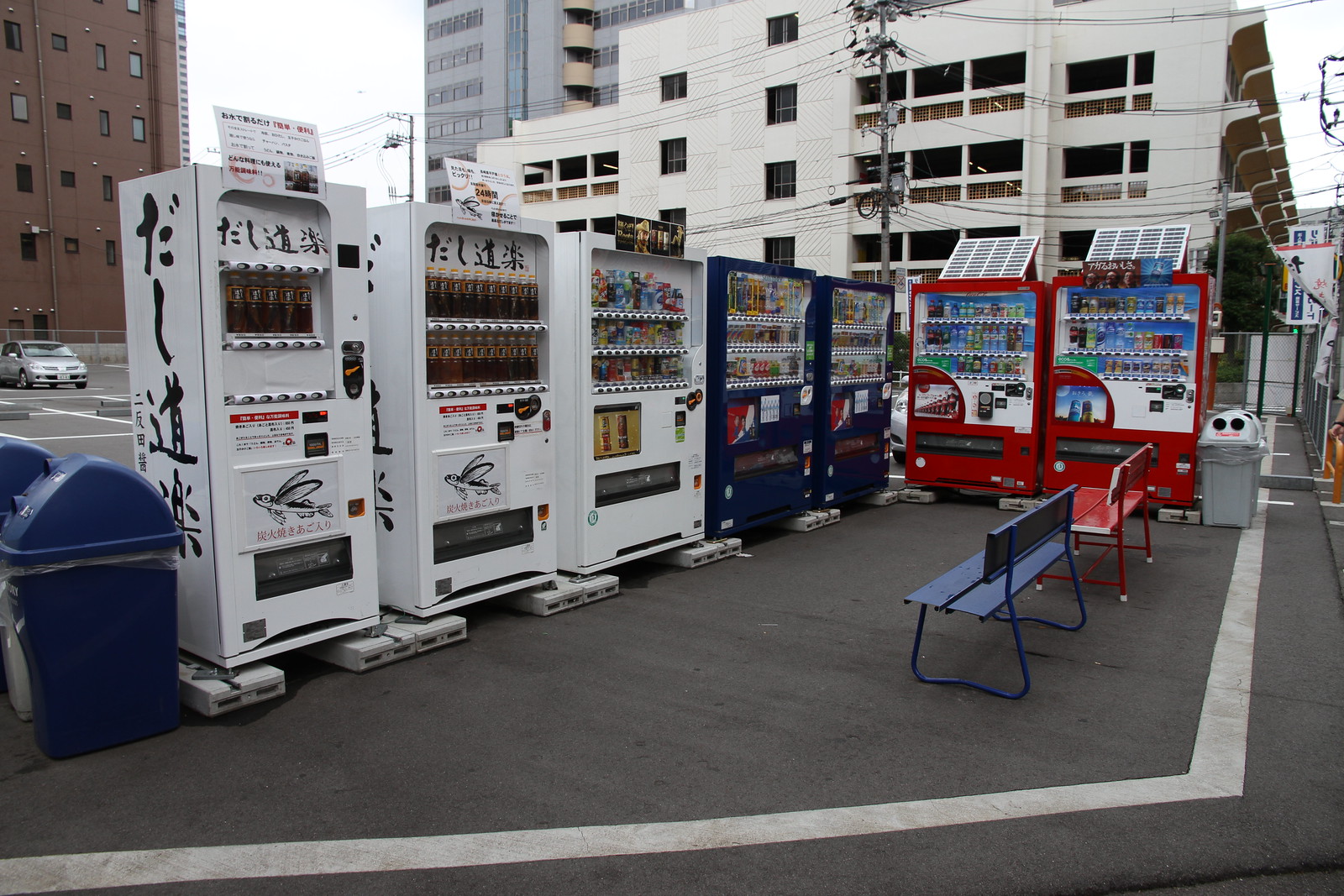This photograph captures several vending machines arranged in an L-formation against a backdrop of various buildings on an overcast day. On the left, three white vending machines feature Japanese text that is not fully legible. The left two white machines also display an image resembling a flying fish or a fish lure just above the dispensing area. Moving to the right, two dark blue vending machines, which likely contain drinks, feature a red, white, and blue logo that appears to be the Pepsi logo, though it's somewhat unclear due to the small size. Continuing to the right, two red vending machines with white details and circular inserts suggest they're selling bottled drinks, though the specifics are difficult to discern.

In front of these vending machines sit two metal benches, one painted blue and the other red, facing toward the machines rather than out to the street. On the far left of the image, a silver car is visible in a mostly empty parking lot, with a large brown building featuring many small windows situated behind it. To the right of the vending machines, there is a gray garbage can marked with two circular openings and a red line. The scene unfolds on dark asphalt, adding to the urban feel of the setting. A large white building, potentially a parking structure or abandoned building with hollow windows, is visible in the background on the right, along with a significant gray building further towards the center.